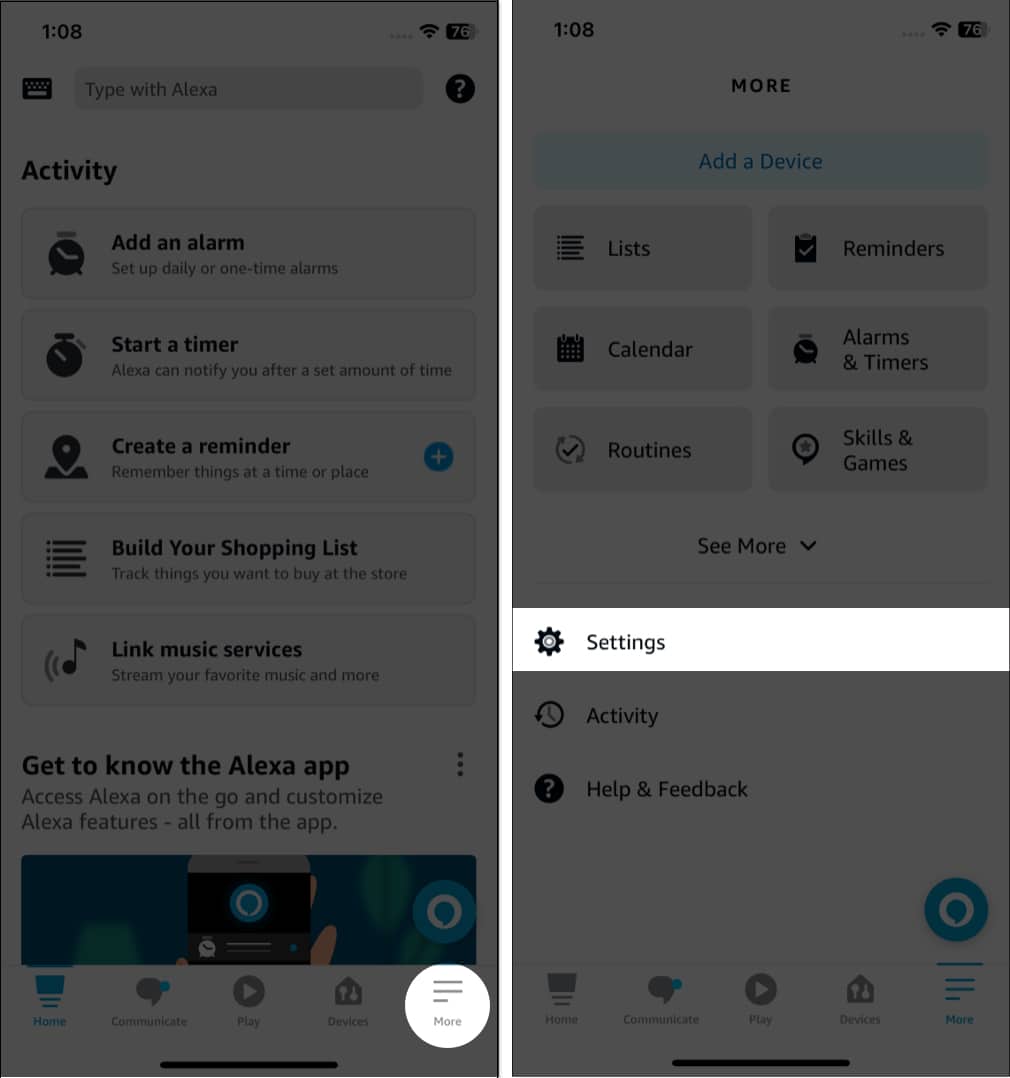The image depicts two interfaces on separate screens, both set against a gray background. 

### Left Screen:
- **Top Left Corner:** Displays the time, "1:08."
- **Top Right Corner:** Contains icons for Wi-Fi and battery percentage.
- **Header:** The text "Type with Alexa" is centered in the middle.
- **Icons Adjacent to Header:** 
  - **Left Side:** Keyboard icon.
  - **Right Side:** A circle icon with a question mark in the center.
- **Sections Listed Below Header:**
  1. **Add an Alarm**
  2. **Start a Timer**
  3. **Create a Reminder:** Accompanied by a small blue circle with a plus sign to its right.
  4. **Build Your Shopping List**
  5. **Link Music Services**
  6. **Get to Know the Alexa App:** Includes a description stating, "Access Alexa on the go and customize Alexa features all from the app."
- **Design Elements:**
  - Below the listed sections is an area designated for further design elements.
  - At the bottom, there are a couple of tabs.
  - A white circle with three lines marked "More."
  - A thin black horizontal bar is positioned centrally at the bottom.

### Right Screen:
- **Top of the Screen:**
  - **Header:** "More."
  - **Blue Rectangle:** "Add a Device."
- **Two Rows of Options:**
  - **Left Column:** Lists, Calendar, and Routines.
  - **Right Column:** Reminders, Alarms and Timers, and Skills and Games.
- **Below the Rows:**
  - Sections titled Settings, Activity, Help, and Feedback.
  - At the very bottom, five categories are displayed, aligning with the rest of the cell phone screen layout.

### Divider:
- The two screens are separated by a small vertical white line.

This detailed caption captures all the elements and their positions as described in the image.